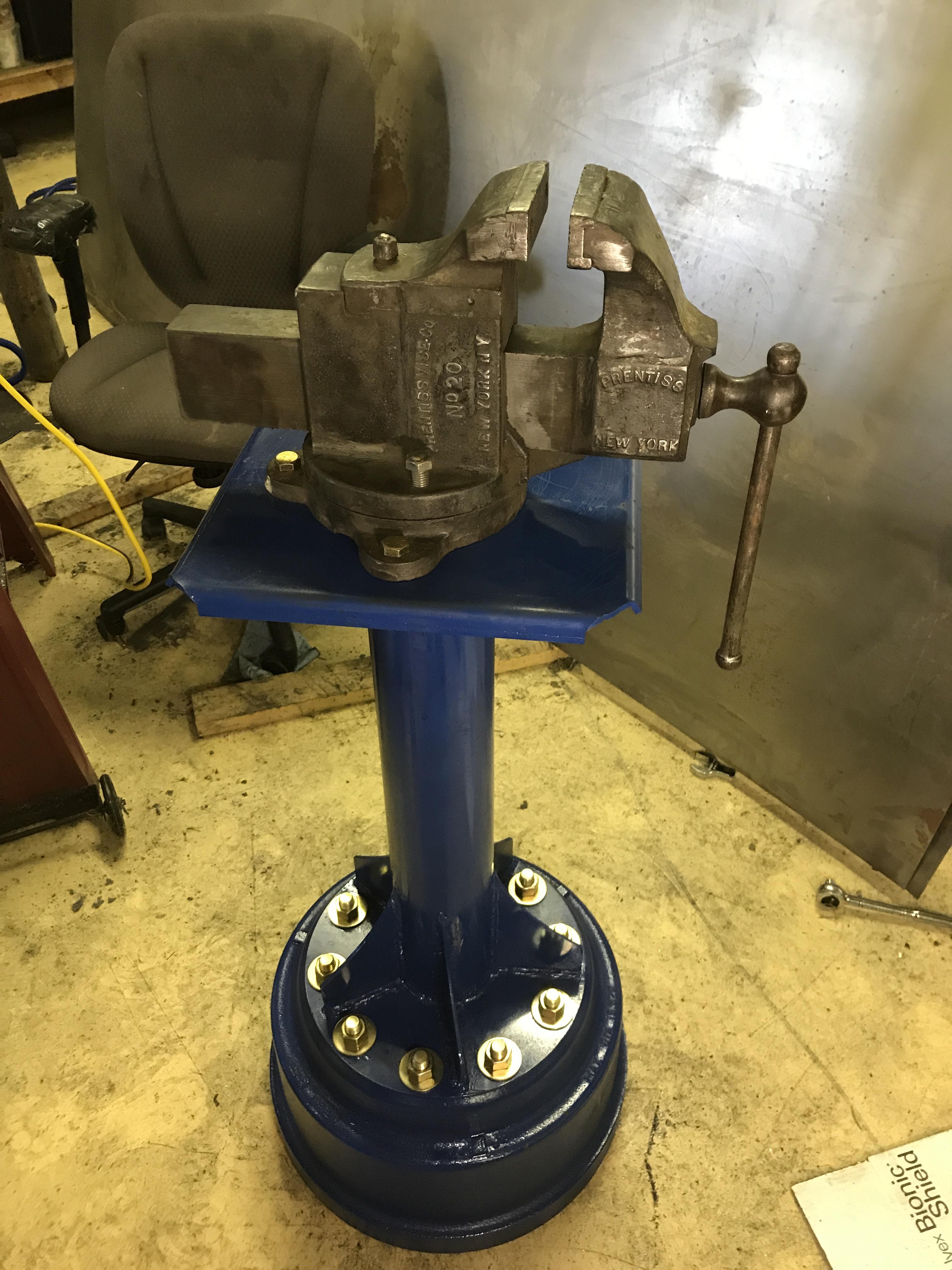The image depicts a large, dark gray steel vise grip mounted on a blue, circular steel pedestal, which is bolted permanently to an old, yellowish linoleum floor. The vise grip, slightly rusted at the top, features a lever on the right-hand side for tightening and loosening. In the foreground, various tools such as a socket wrench and a regular wrench are strewn about, alongside a white sign. To the left, there are wheels that appear to belong to a tool cabinet. In the background, an old, gray office chair with a ragged left side is visible, set against a rust-spotted steel wall. Additionally, a yellow cord and the bottom portion of a dark red stand can be seen in the vicinity of the chair. A wooden shelf is partially visible, shrouded in shadow behind the steel wall, contributing to the industrial or garage-like ambiance of the setting.